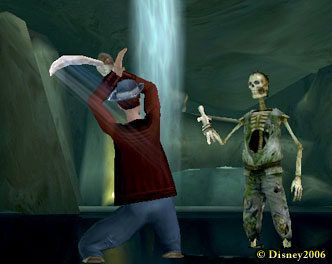This image is a screenshot from the now-defunct Disney MMORPG, Pirates of the Caribbean Online. The scene is set inside a dimly lit cave with intricate gray rocky formations. A striking waterfall cascades down the center, its light blue waters falling about two-thirds of the way down the screen. The rocky surroundings form an elaborate backdrop.

In the foreground, to the left, stands a pirate character with his back to the viewer. He wears a blue hat atop short brown hair, a red long-sleeve shirt, blue pants, and visible boot tops. His left arm extends outward while his right hand, bent at the elbow, raises a long silver pirate scimitar, poised to strike. His posture suggests he's about to attack the menacing skeleton figure positioned across from him.

The skeleton opponent, located on the right side of the image, is dressed in a tattered gray shirt and pants with patches of moss. The skeletal figure has an exposed ribcage and hollowed stomach area, emphasizing its undead state. One bony arm extends, clutching a voodoo doll, while the other arm dangles by its side.

The characters are ankle-deep in water, adding to the eerie atmosphere. In the bottom right corner of the image, the yellow text reads "Disney 2006," confirming the age and origin of the game.